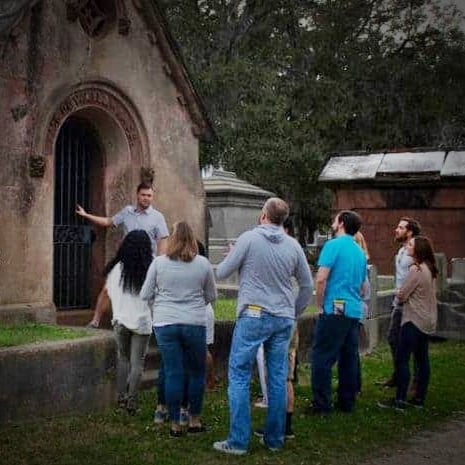The photograph portrays a tour group gathered around an old mausoleum within a cemetery. The structure, made of aged stone with a light brown coloration, features a moss-covered exterior and an arched doorway adorned with unreadable writing. A man, likely the tour guide, stands on a few steps leading up to this grand entrance, extending his hand towards the mausoleum's iron gate. He is dressed in a blue short-sleeved button-down shirt, distinguishing himself from the casually dressed participants, who are mostly wearing grayish shirts and denim jeans. The group of six or more people forms a semicircle on the grass, attentively listening, some with pamphlets visibly tucked in their back pockets. In the background, the scene is framed by tall, leafy green trees and a low-lying building, possibly a shed with an old gray roof, adding to the historical ambiance of the setting. The weather appears overcast, casting a slightly gloomy atmosphere over the tour.